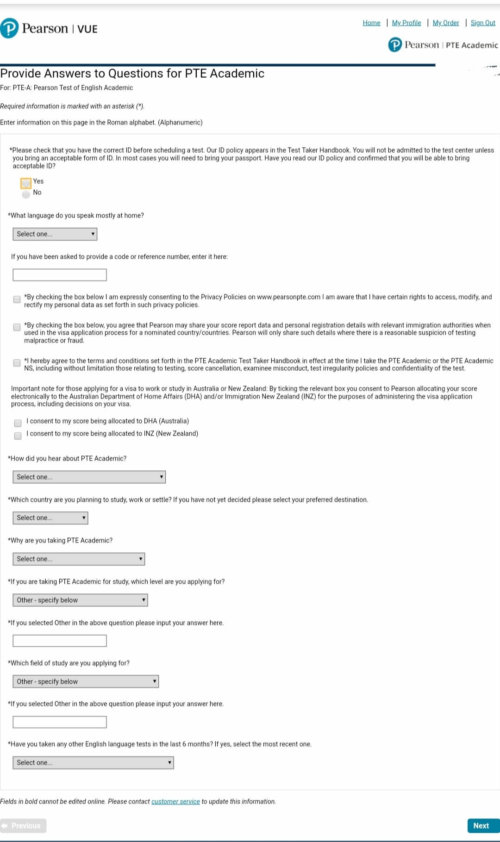Screenshot of the Pearson VUE webpage, showing the following details:

- **Top Navigation Bar:**
  - At the top left, there's a "P" logo followed by the text "Pearson VUE" in black.
  - On the far right, there are a series of hyperlinked text options: "Home," "Wishlists," and two additional links in small blue writing.

- **Main Header:**
  - Below the navigation bar, the Pearson logo appears again alongside the text "Pearson PTE Academic."
  - This section is separated from the rest of the content by a black horizontal line.

- **Body of the Page:**
  - Just below the black line, at the top left, the heading "Provide answers to questions for PTE Academic" is displayed in bold black letters.
  - Below this heading, there's smaller, harder-to-read text, including the phrase "PTEA Pearson."

- **Main Content:**
  - The central part of the page consists of a series of questions accompanied by drop-down boxes for selecting answers, extending down the length of the page.

- **Footer:**
  - At the bottom right corner, a blue button labeled "Next" is visible.